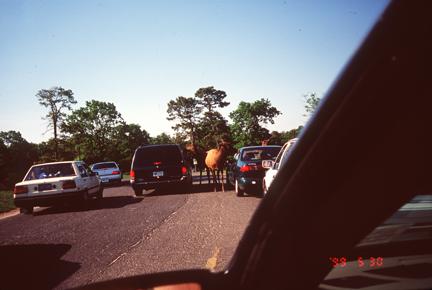This photograph, likely taken on May 30, 1999, as indicated by the watermark "99 530" in the bottom right corner, captures a scene at the entrance to what appears to be a park, possibly a zoo or safari park. The image shows a three-lane roadway where multiple vehicles are halted. Each vehicle is interacting with a uniformed individual who appears to be facilitating entry. Notably, there is a Chrysler van present among the vehicles. Adding an intriguing element to the scene, two moose can be seen, seemingly involved in the process, instead of a person as initially thought. These moose contribute a unique and unexpected aspect to the photograph, marking the entrance as being in a wildlife-related facility.